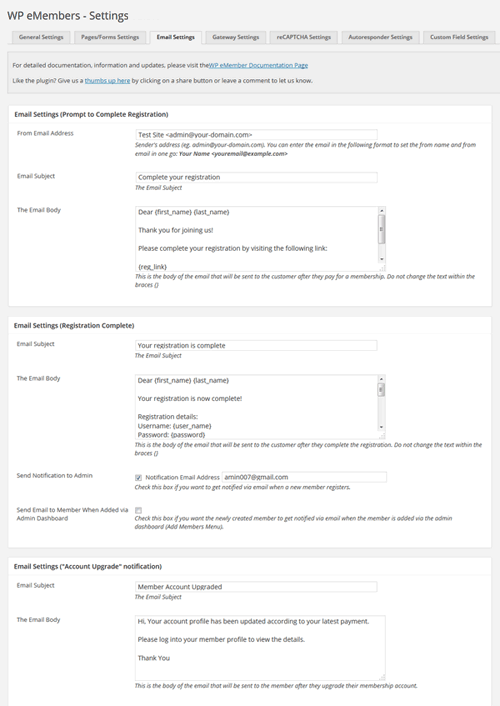This image showcases a webpage interface, primarily focused on the WP e-Members settings section. The website header spans about an inch and a half and is colored in light gray. Flanking both the left and right sides of the webpage is also a light gray border. Below the header, there is a narrow segment transitioning into a white background with thin gray borders repeating horizontally twice, each about two inches wide, before extending further down the page into a continuous white background.

On the top left corner in bold black text is the title, "WP e-Members Settings." Directly beneath this title are seven navigable tabs displayed horizontally. These tabs are gray with light gray text, except for the third tab, which stands out in white with black text, indicating it is the active tab.

Below the tabs, there is a blue hyperlink labeled "Member Documentation." Continuing downward, another line features a blue thumbs-up icon. The next section displays "Email Settings" in bold black text followed by "Prompt to Complete Registration." Underneath, it provides instructional details on how to execute this process.

Further down, a white rectangular box is labeled "Email Settings (Registration Complete)," containing sections for "Email Subject," "Email Body," and other related fields. The final segment at the bottom of the image presents another section titled "Email Settings (Account Upgrade Notification)," which also includes areas to fill in the "Email Subject" and "Email Body."